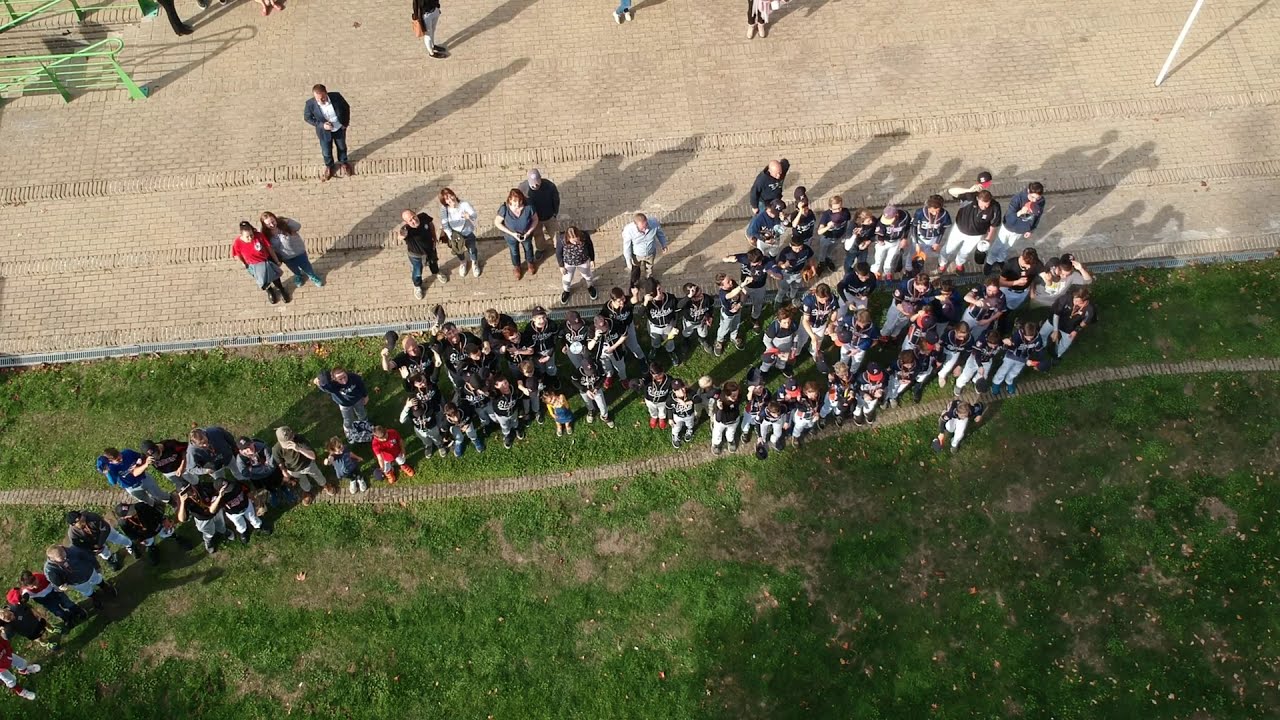This is an overhead photograph showcasing a large gathering of over 50 people on a grassy lawn. The crowd includes children and adults, many of whom are dressed in matching black baseball shirts and hats, suggesting they might be a team. They are standing in a line, facing towards the bottom of the photograph, possibly posing for a picture. Behind them, a brick walkway or entryway, complete with steps, is filled with additional onlookers. Some people in the crowd are pointing upwards towards the camera. In the left corner of the image, a bright green metal staircase is visible, while the upper part of the photo shows people's feet, indicating a larger crowd beyond the frame. The bottom part of the photograph shows a grassy area with a narrow pathway weaving from left to right amidst the gathering.